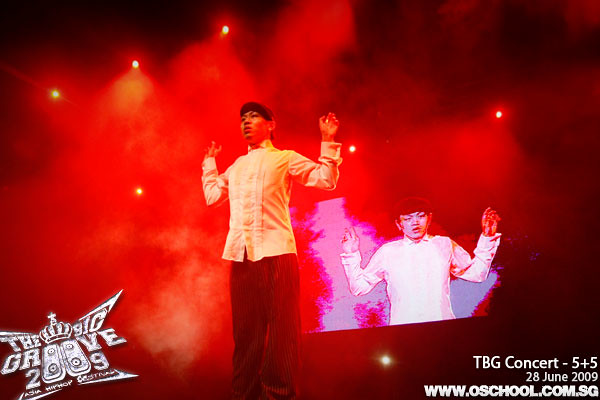In this vibrant photograph, a man stands center stage, exuding energy and poise with his arms extended in a dynamic V shape. He is smartly dressed in a white dress shirt and dark slacks, accessorized with a stylish hat, suggesting a performer in the midst of an engaging act. The backdrop features a large screen displaying "The Big Groove 2009, TBG Concert 5 plus 5, 28 June 2009, www.oschool.com.sg," with text visually striking like silver-studded diamonds. The scene is indoors, marked by the glow of overhead stage lights that enhance the colors of the image—black, red, white, gray, purple, and blue—creating a lively and thrilling atmosphere. The meticulous arrangement of elements and the performer's central position highlight the intense and captivating nature of the concert. In the lower left, a crown-like logo emphasizes the grandeur of the event, further immersing the viewer in this energetic and memorable performance.